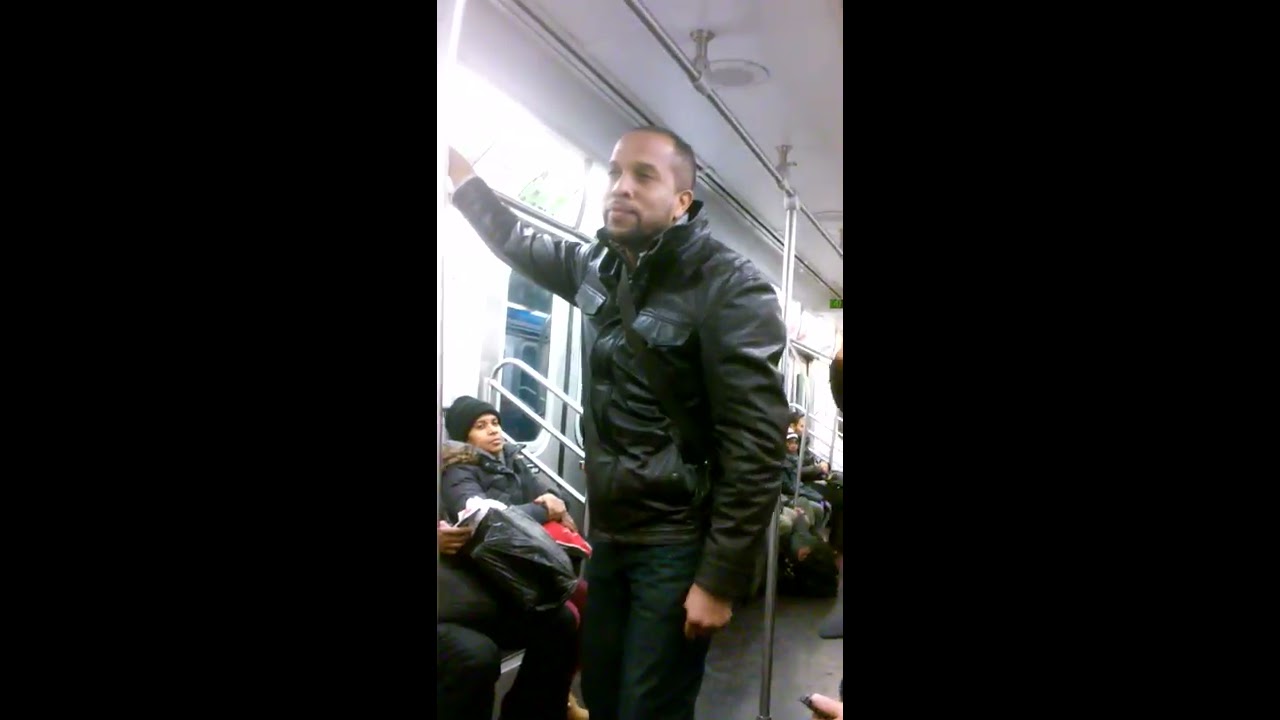This full-color photograph, taken during the daytime inside a New York subway, is horizontally rectangular with very thick black borders on both sides, framing a vertically rectangular center panel that captures the actual scene. The primary focus is a young black man with light brown skin, standing and holding onto a metal pole. He is dressed in a black leather jacket that is fully zipped up and dark blue jeans, with a bag slung over his shoulder. His neatly trimmed goatee is visible as he gazes off into the distance to the left, his eyes clearly seen in the image. His right arm is raised, clutching the pole on the top left corner of the photograph, while his left arm rests at his side in a fist. Behind him, slightly to the left near the subway doors, a woman in a dark blue puffer jacket and a black hat is seated, holding a red object, and appears to be gazing in the direction of the camera. The light filters through the subway windows, illuminating the scene and highlighting the various passengers who occupy the background seats.